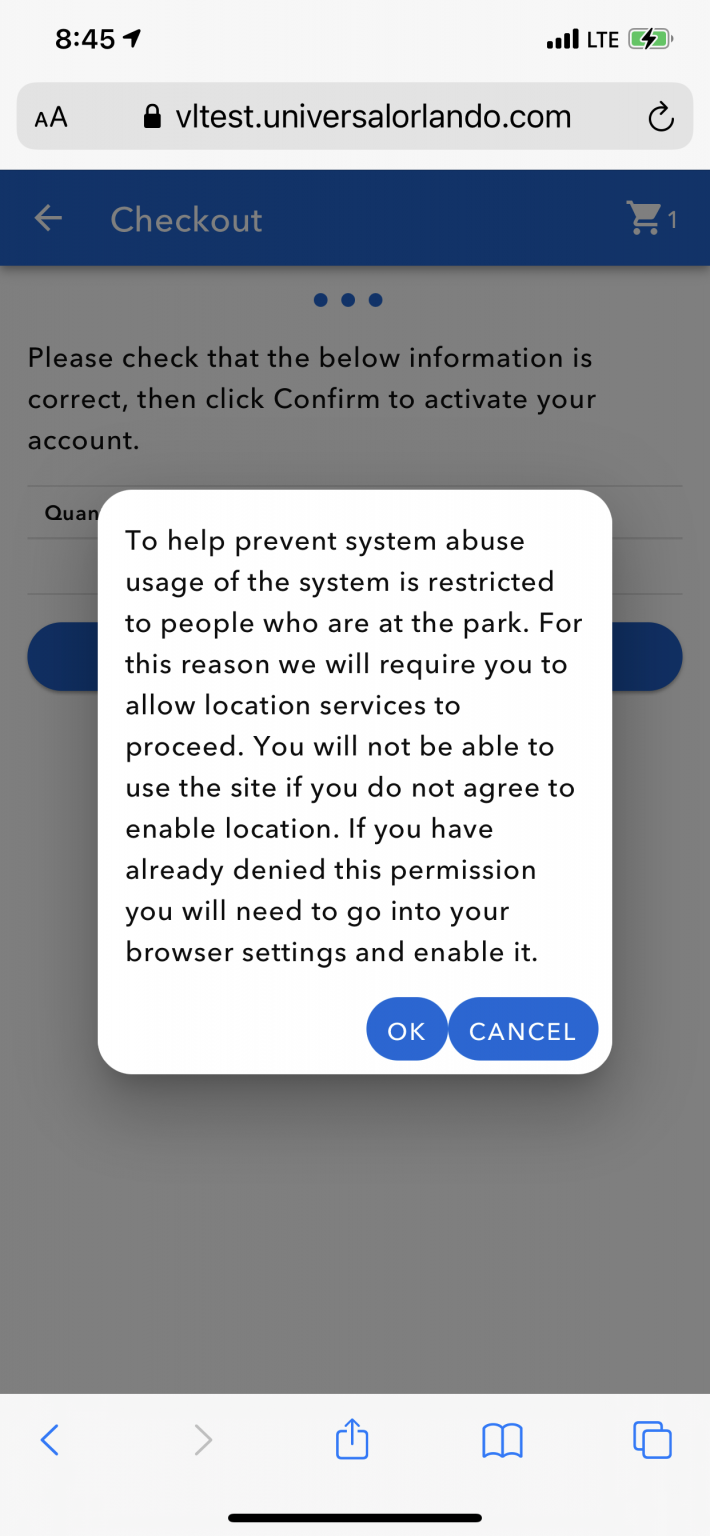The image appears to be a screenshot from a mobile phone. At the very top, there is a gray status bar displaying the time as 8:45, along with four signal bars, "LTE" indicating cellular network type, and a green battery icon. Below this, a gray browser navigation bar is visible, showing a padlock symbol, the URL "vitest.universalorlando.com," and a refresh icon.

Beneath the browser bar, a blue section with the text "Check Out" accompanied by a shopping cart icon can be seen. Following this, there is a white section instructing users to verify their information: "Please check that the below information is correct. Then click Confirm to activate your account." 

A prominent white pop-up box appears in the middle of the screen with a detailed message, stating that to prevent system abuse, the service can only be used by individuals located in the park. It explains that location services need to be enabled for continued use. The message advises users on how to enable location services if permission has already been denied.

This pop-up features two buttons at the bottom: a blue circular button labeled "OK" and a blue oval button labeled "Cancel." The background of the image below the pop-up box is largely blank.

At the very bottom of the phone screen, a navigation bar displays icons for back navigation (a left-pointing arrow), downloading (a downward arrow), viewing bookmarks (a book icon), and managing open tabs (an icon resembling two overlapping squares).